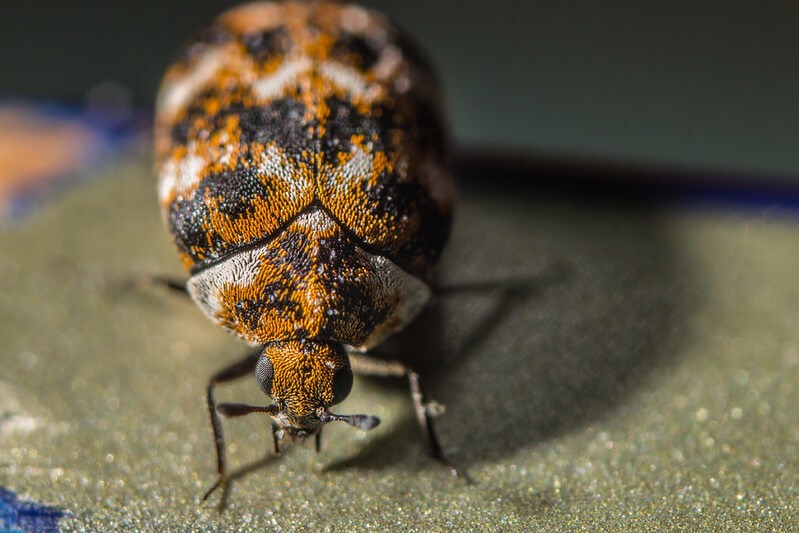This image is an extreme close-up of a beetle-like insect situated on a surface that appears to be either a grayish, grainy floor tile or a leaf. The backdrop is blurred, featuring diffuse hues of blue, orange, gray, and green. The insect occupies a position slightly left of center in the vertical rectangular frame, facing towards the camera. It's primarily dark orange with prominent black spots and intricate white jagged lines horizontally traversing its oval body. The beetle’s head, smaller in size, is dark orange with noticeable black circular eyes and extends two black antennae. The insect has four visible legs—two in the front and two in the back. The texture of its body suggests a scale-like or finger-like pattern, adding to the detailed visual complexity of its exoskeleton.